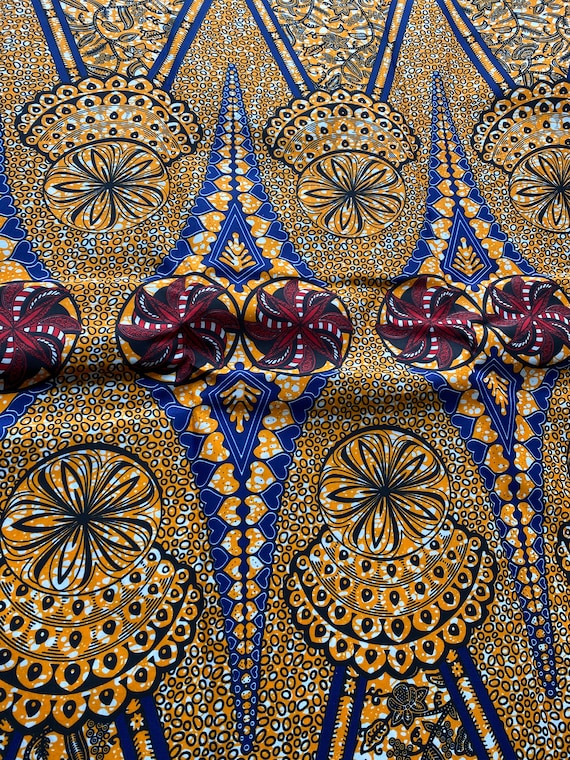This vertical rectangular image showcases a piece of intricately designed fabric that is laying flat, but with a subtle outline in the middle suggesting something, perhaps a drawer handle, lies underneath. The fabric is resplendent with a rich tapestry of vibrant colors including blue, red, yellow, black, and white. Dominating the design are two elongated blue diamond shapes embellished with golden heart motifs arranged back-to-back along the edges. The heart motifs ascend and descend continuously along the fabric, adding an element of rhythm. Between these diamonds, two circular patterns stand out, adorned with red pinwheel designs, each of which is dotted with white along its arms. These circles also encompass lace-like elements beneath them, suggesting delicate intricacy. Additionally, the design incorporates ribbons and bead-like bands, and within some circles are petal or leaf-like shapes, evoking an African tribal aesthetic. The fabric fills the entire frame, creating a visually engaging and warm presentation, hinting at the thought that it may be concealing something beneath.